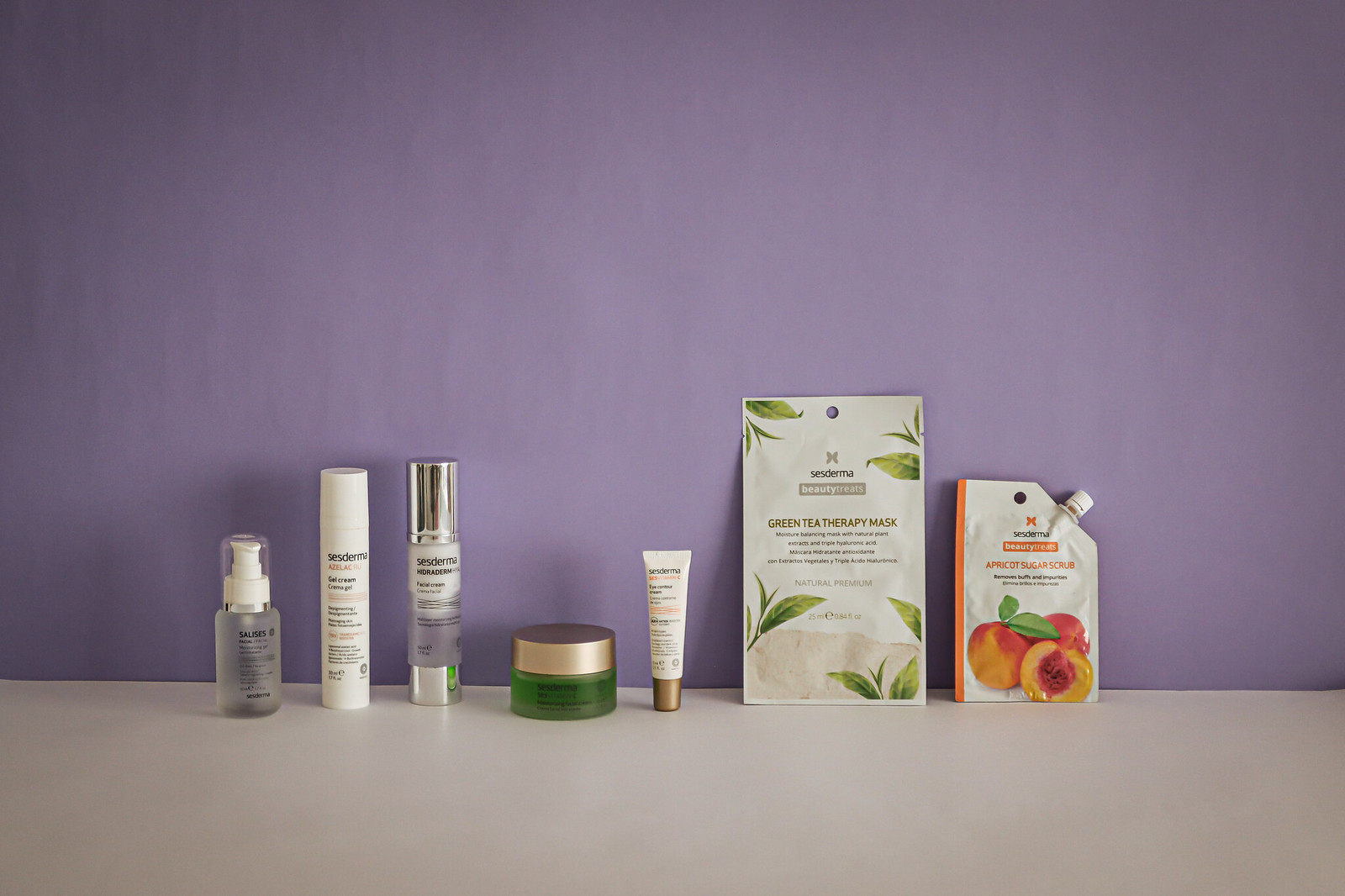A neatly arranged selection of skincare products is displayed against a soft lavender background, reminiscent of a painted wall. The items rest on a light gray table, creating a subtle yet elegant contrast. To the right side, a variety of Acesderma Beauty Treats products are clearly visible, including an Apricot Sugar Scrub and a Green Tea Therapy Mask. In addition to these, there is a sleek tube adorned with a silver cap, a solid white tube, a cylindrical container featuring a green base, and another tube equipped with a convenient pump. The consistency in design and branding suggests that all these items belong to the same product line, emphasizing a cohesive and sophisticated skincare collection.